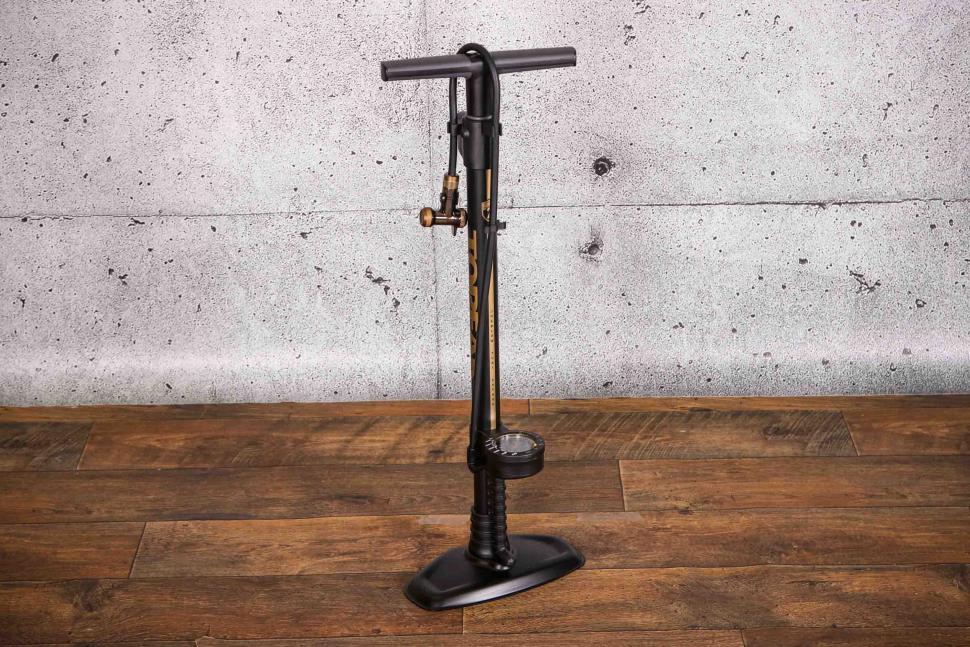The image showcases a black bicycle air pump standing upright on a wooden, paneled floor. The pump, resembling a pogo stick in shape, includes a black handle and base. The main body of the pump features gold branding and lettering, with a gold-colored nozzle at the end of the hose. The air pressure gauge is situated near the base, allowing for easy monitoring while inflating tires. The hose extends from the bottom and wraps around the handle. The background consists of four large concrete blocks divided into rectangles, creating a greyish, speckled wall. The pump is slightly angled, with the left side closer to the foreground of the image.